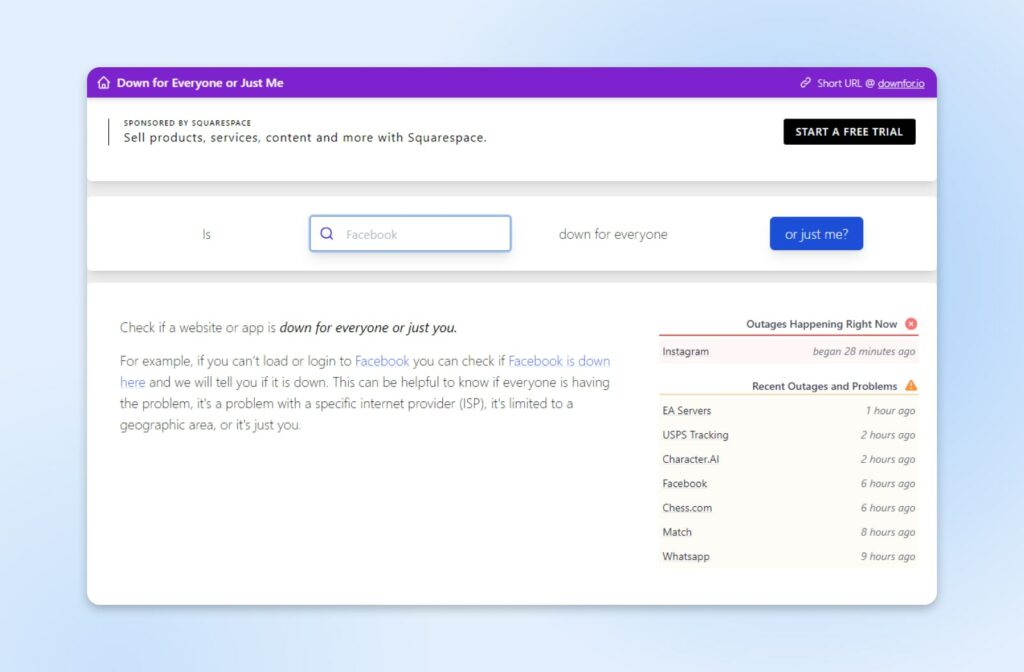Screenshot of an online tool for checking website statuses. The webpage prominently features a heading in purple that reads "Down for Everyone or Just Me," indicating its purpose—to help users determine if websites are universally down or if the issue is isolated to their own connection. Below the heading, there are two links, though the smaller text is not clearly legible. A notable "Free Trial" button is also visible, suggesting the availability of additional features upon subscription.

Users can input the URL of the website they wish to check into a designated search bar—Facebook is used as an example in this instance. By clicking the "or just me" button, the tool initiates a status check. On the right side of the interface, there's a list providing real-time updates on currently active outages. For example, it notes that Instagram has been experiencing issues for the past 28 minutes. The list continues with recent outages and problems from other websites, documenting occurrences from an hour ago or more.

The overall design is clean and functional, offering users a straightforward method to verify website accessibility and troubleshoot potential connectivity issues.